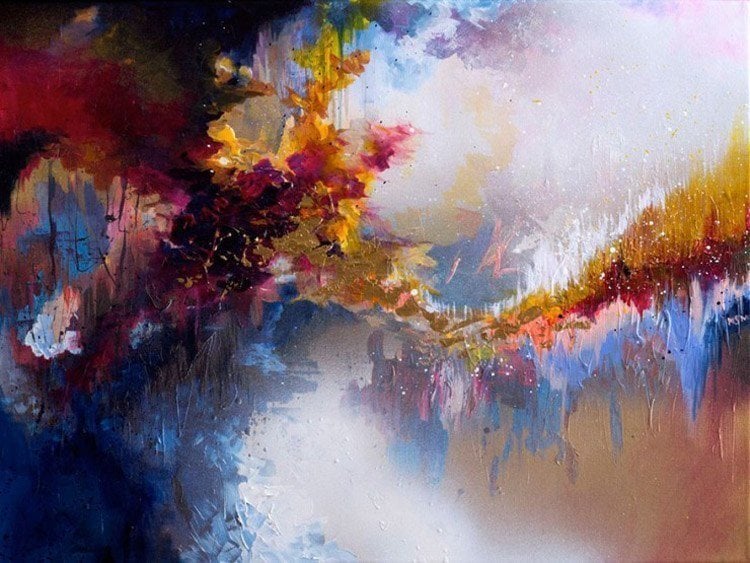This wide rectangular image appears to be an abstract digital art piece, potentially evoking a painting. The composition showcases a myriad of vibrant colors and textures, reminiscent of splattered paint or a dynamic natural scene. On the right side of the image, both the bottom and top corner sections feature white spaces, interspersed with hints of sky blue, a pale tan, and violet. A striking yellowish-gold segment runs horizontally through the middle, transitioning into a trail of goldish brown that extends to the right edge and ends in pink and gold.

The left section of the image is predominantly darker, with a mix of black, red, and green. Beneath this area, there are splashes of blue, pink, and speckled white, which then shift back to darker shades of black and blue towards the middle. The middle section begins to lighten with colors such as white, sky blue, gold, mustard, and pink, creating a vibrant and varied palette. Throughout the piece, there are recurring hues of red, blue, orange, and purple, giving the artwork a vivid, almost seasonal appearance. Without any text or artist attribution, the piece remains anonymous but captivates with its unique and visually intriguing design.